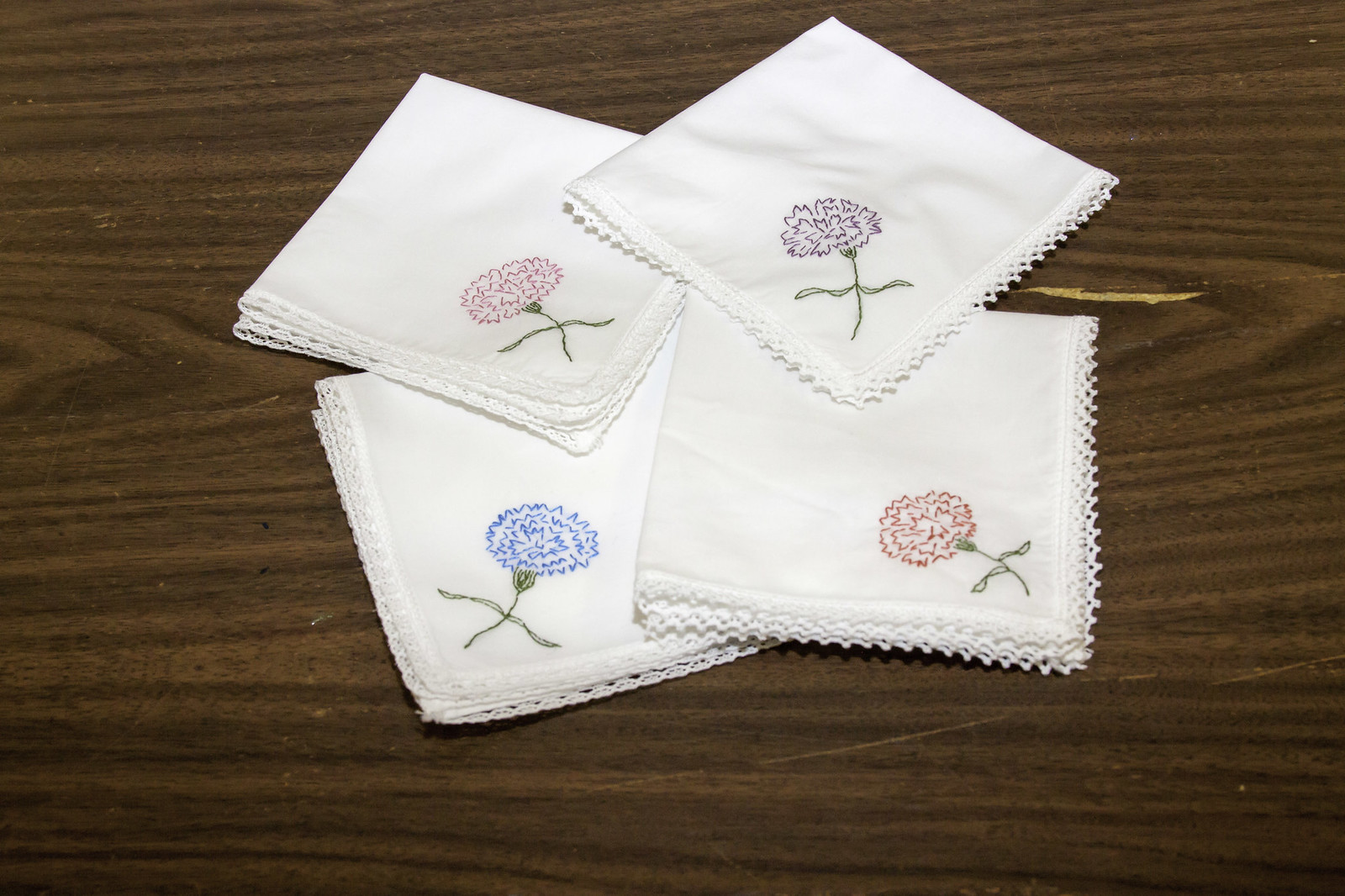The image features four intricately embroidered white cloths, likely handkerchiefs or large napkins, each carefully folded into quarters and displayed in a staggered pile on a dark, aged wood grain surface, exhibiting visible cracks and signs of wear. The ornate edging of the cloths is elegantly serrated, and the beautiful, simple embroidery is positioned in the corners of each folded piece. The embroidered designs consist of colorful flowers with green stems and leaves, possibly resembling carnations, bachelor's buttons, or other dianthus species. The flowers are depicted in distinct colors: pink, deep purple, blue, and red. Despite the overlap in the stacking arrangement, each embroidered flower remains visible, enhancing the overall aesthetic appeal of this meticulously presented set.